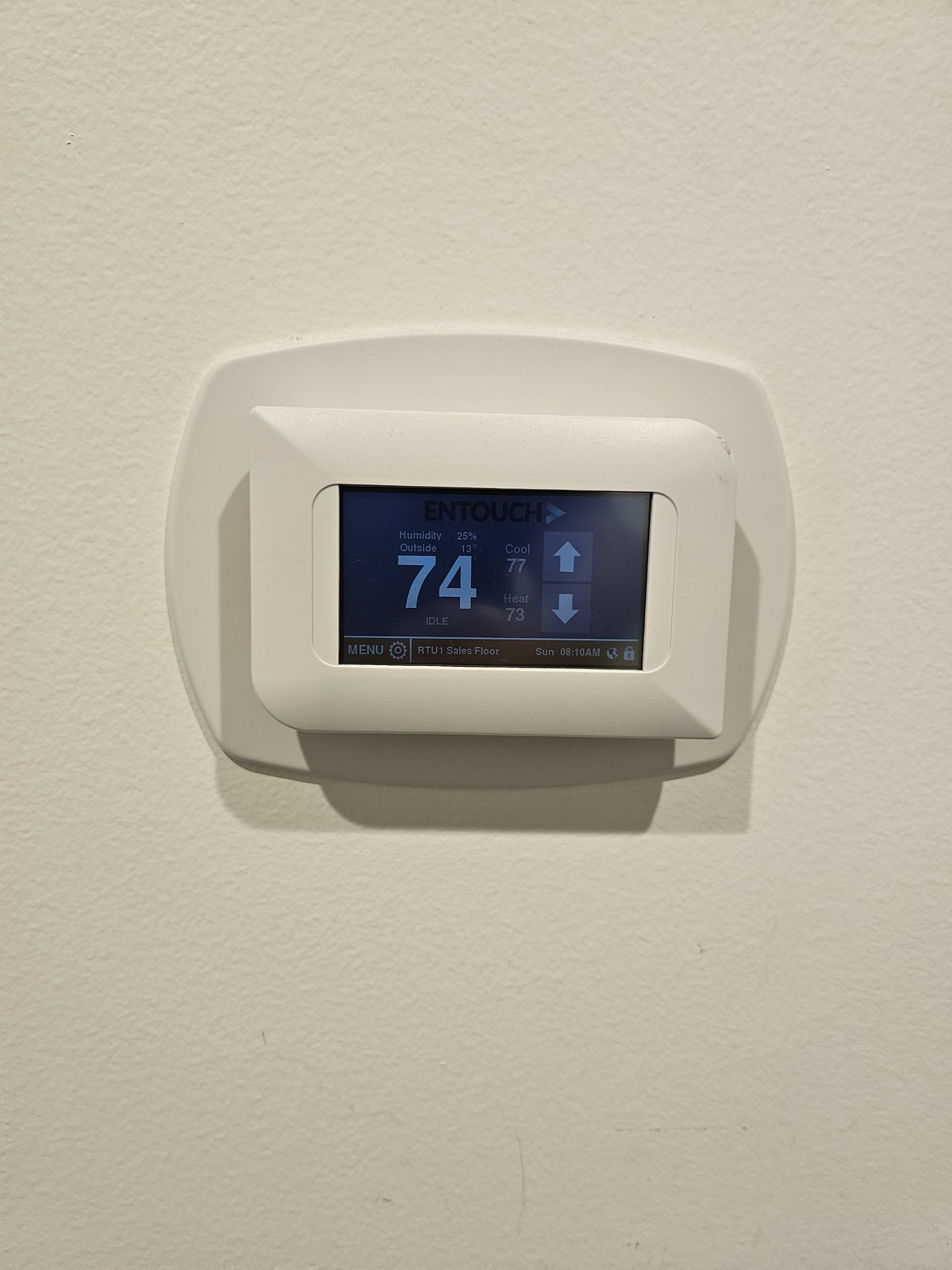A face-on photograph captures a thermostat or temperature regulator crafted from cream-colored plastic, centrally mounted on a matching cream plastic base. Both elements are affixed to a cream-painted wall featuring a rough texture. The wall shows slight wear, with minor scuffs visible in the bottom right-hand corner. The thermostat, prominently positioned in the middle of the frame, boasts a sleek, curved design that rises from the base. Its dark blue screen displays the temperature in bold, pale blue numbers reading "74°F." Adjacent to this are temperature range indicators showing "77°F" and "73°F," flanked by two pale blue arrows stacked vertically. Beneath the screen, a black strip holds text including "menu," additional smaller text, the day "Sunday," a small internet globe icon, and a lock icon.